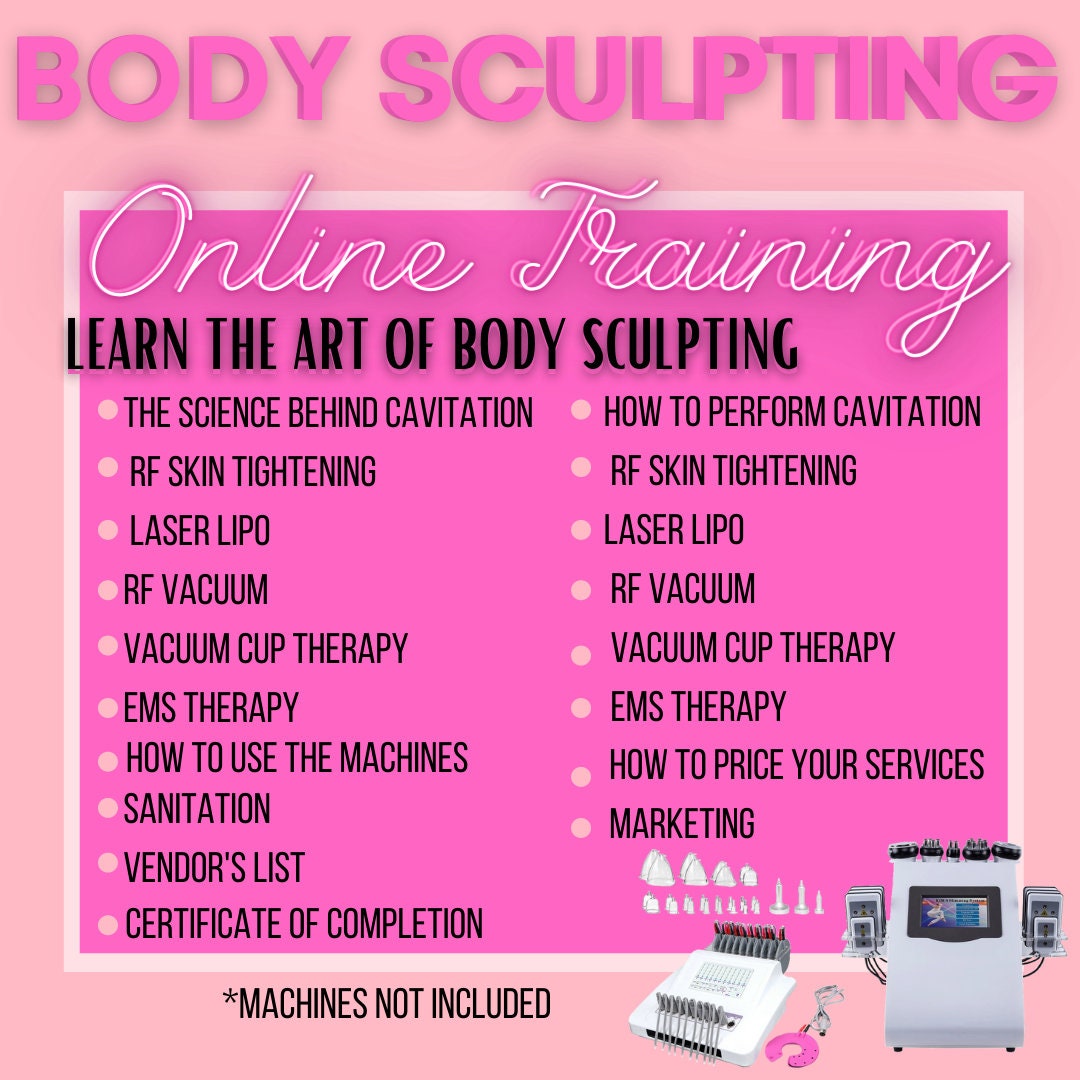This poster is an advertisement for an online body sculpting training class, prominently featuring a pink-themed design. At the top, the words "Body Sculpting" are written in large pink letters. Below, a bright pink square centered on the flyer contains the text "Online Training" in white cursive lettering, followed by "Learn the Art of Body Sculpting" in black letters. Underneath, there are several white bullet points organized into two columns. The left column lists: the science behind cavitation, RF skin tightening, laser lipo, RF vacuum, vacuum cup therapy, EMS therapy, how to use the machines, sanitation, vendors list, and certificate of completion. The right column states: how to perform cavitation, RF skin tightening, laser lipo, RF vacuum, vacuum cup therapy, EMS therapy, how to price your services, and marketing. At the bottom right, there are images of white machines used for body sculpting, accompanied by the note "machines not included" in black text.